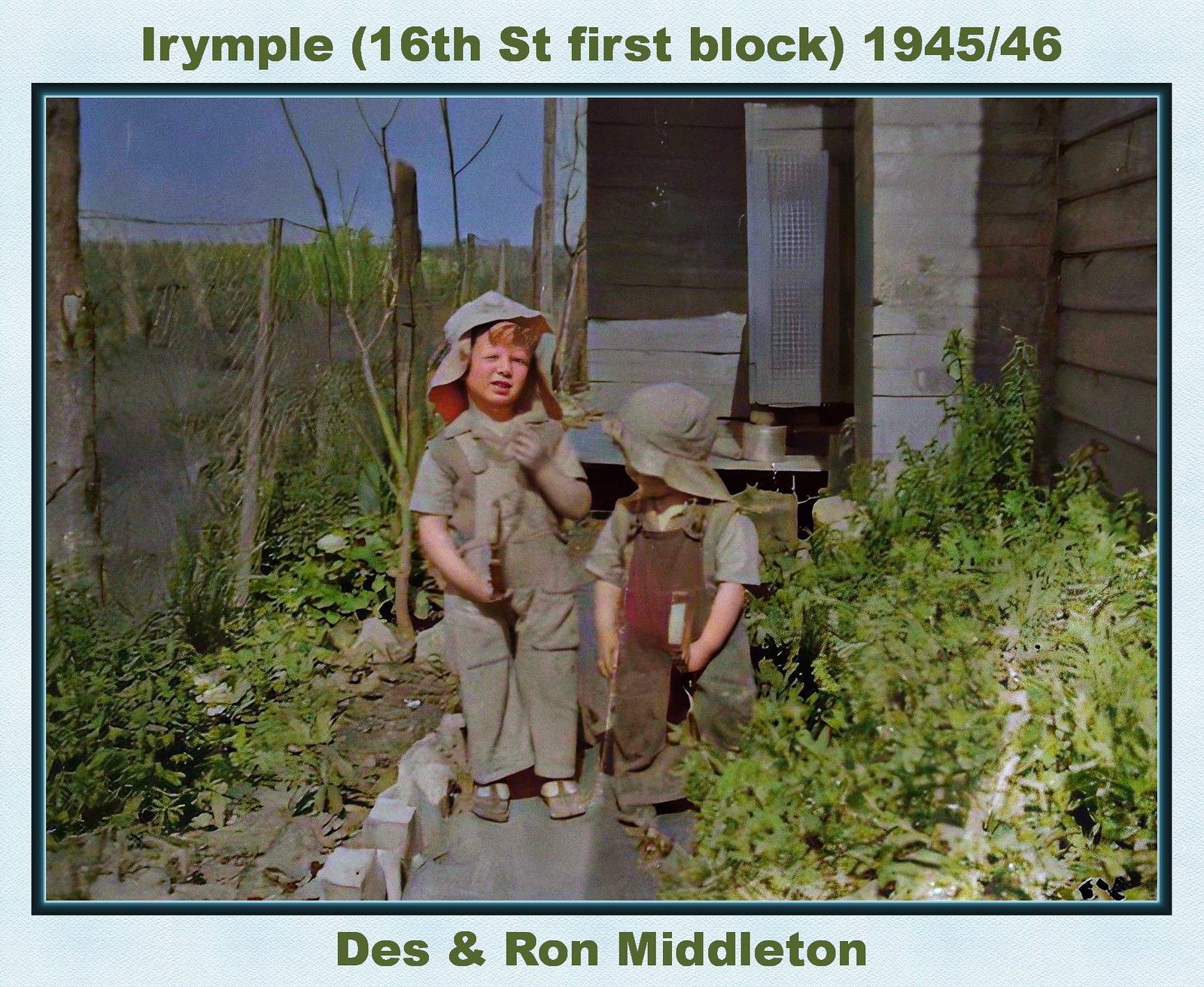This is an old, professionally-taken photograph from 1945-46 captioned "Irymple, 16th Street, 1st Block" at the top in green and "Des and Ron Middleton" at the bottom, also in green. The image features two young boys, Des and Ron Middleton, standing on a walkway leading up to a house. The taller, older boy on the left has red hair, a pink face, and is squinting his eyes against the bright sun. Both boys are dressed in matching brown or khaki overalls paired with little shirts, sandals, and wide-brimmed, floppy hats for sun protection. The younger boy on the right has his face turned away from the camera, making it difficult to see his features. The scene includes a surrounding landscape of grass, dirt, and vegetation, with a wire fence to the left and more plant life and a glimpse of the house with visible shingles behind them. The overall setting suggests a front yard of a rural home, with signs of a small concrete walkway bordered by bricks and shrubbery.